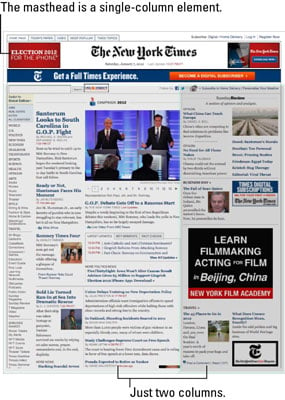The image, sourced from the New York Times, prominently features the publication's masthead in bold black print. At the top of the page, a clear indication refers to the masthead as a "single column element." Below it, a highlighted section marked with a red box reads "Election 2012," from which a black line extends to connect back up to the masthead connection point. The page is populated with multiple articles and accompanying pictures scattered throughout, offering a comprehensive visual representation of the news layout. At the bottom, the image depicts a complex structural layout with lines intersecting and connecting, illustrating the division of content into two distinct columns. These columns are specifically indicated with labeled lines pointing to sections on both the left and right sides of the page.